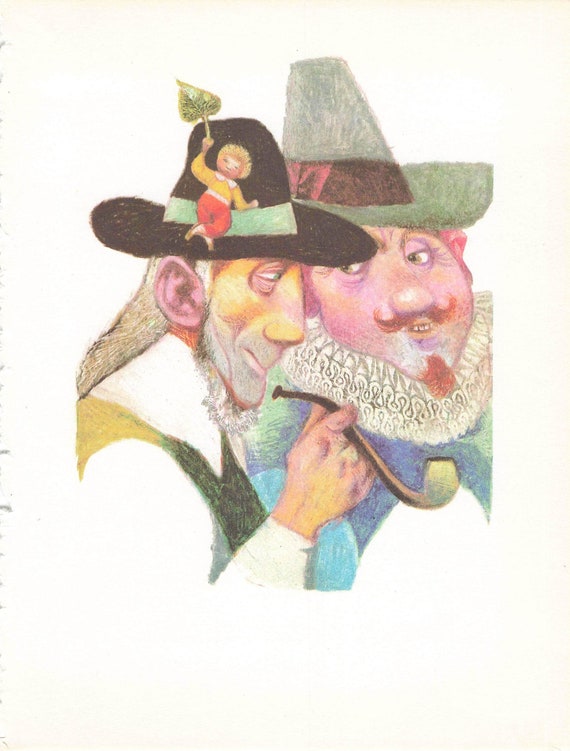The image is a vertically rectangular drawing framed by a light cream border, featuring two cartoonish men who are not in modern-day clothing. The man in the foreground, on the left, has a large black hat with a green ribbon, adorned with a little character (variously described as a baby, little boy, or bear) holding a leaf or three-leaf clover. His skin tones mix orange, yellow, and pink, and he has distinct large ears, a bit of a beard or five o'clock shadow, and puffs on a long-curved stem pipe. He is dressed in a white shirt and a black and brown vest. The second man stands closely behind him on the right, wearing a green hat with an orange or black band. His skin is purple and pink, with a red mustache and goatee, and he sports a lacy collar and a blue shirt. Both men are depicted as if they are happily schmoozing or chit-chatting, giving off an amiable, leisurely vibe. The detailed and vibrant artwork emphasizes their clothing, accessories, and distinctive facial features.